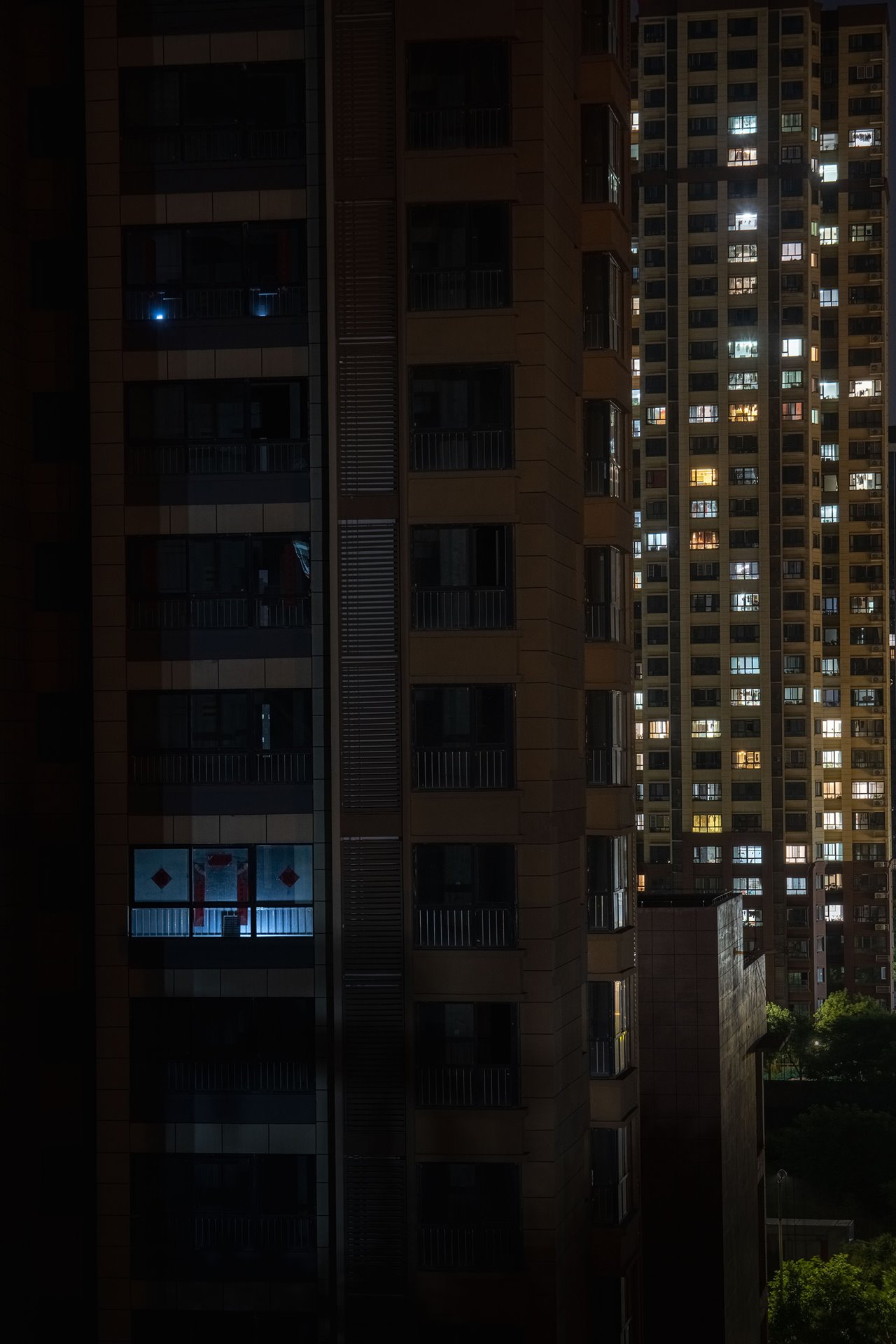This nighttime portrait-oriented image depicts a downtown area dominated by two skyscrapers. The building in the foreground on the left, towering with at least 100 floors, has most of its lights turned off except for one room with a three-panel sliding glass door opening to a railed balcony. This illuminated room emits a pale blue light amidst the darkness. In the bottom right corner, there are some bushes adding a touch of green to the scene. The second building, located further back on the right, is equally tall if not taller. It features numerous illuminated windows scattered across its facade, creating a striking column of intermittent lights. Many floors are bathed in artificial lighting, with some sections notably brighter. Amidst the interplay of light and shadow, both buildings stand out against a backdrop of blackness, showcasing the stark difference between the unlit and illuminated interior spaces.